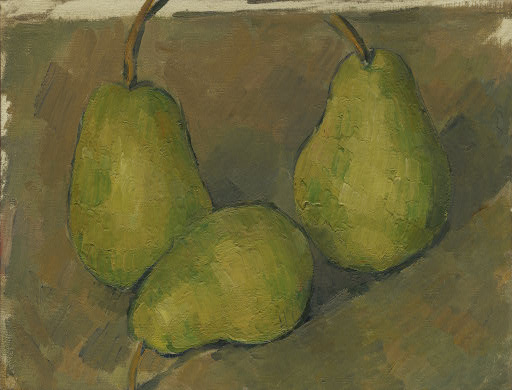The painting, titled "Three Pears" by Paul Cezanne from around 1878, is a detailed still-life oil painting in a landscape orientation that leans towards realism rather than abstraction. It depicts three green pears, rendered with a textured, almost popcorn ceiling-like quality. The pears, with large stems, are set against a background of broad, greenish-brown paint strokes. Two pears stand upright, while the middle pear lies on its side. The pears are highlighted with a slight shine to capture a realistic look, and shadows are visible on the dark green ground, suggesting a nuanced play of light. The background features hints of white, possibly representing a wall or land, painted in shades that emphasize the pears' natural colors and textures. The painting showcases the Impressionism and Post-Impressionism styles characteristic of Cezanne’s work.